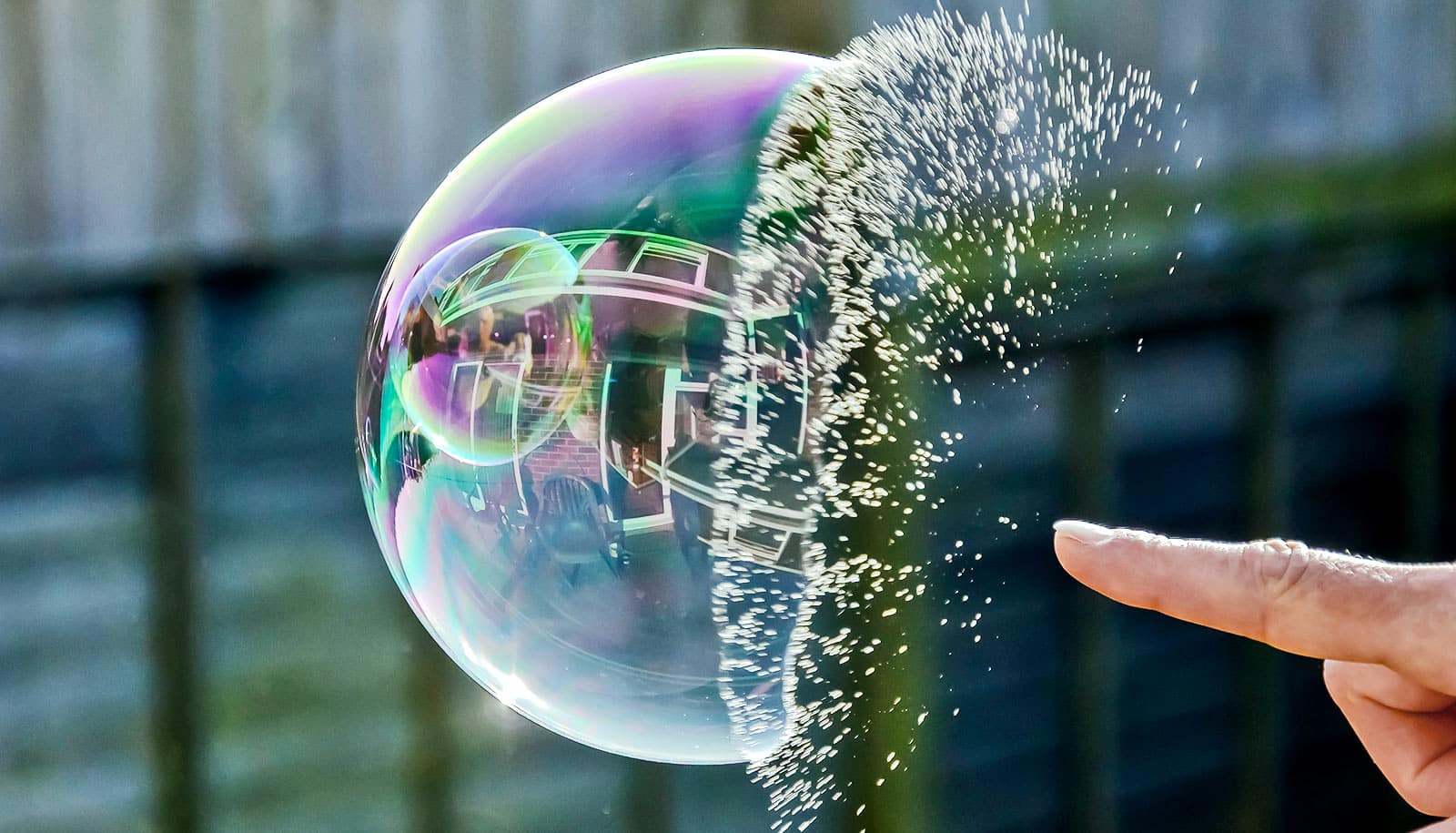In this close-up image, a person is captured in the act of popping a bubble. Emerging from the lower right-hand corner is the side of a hand, prominently featuring an extended index finger pointed straight out towards the bubble. The bubble itself, located on the left side of the image, displays a vivid purple hue. In the moment of contact, the bubble is shown midway through the popping process, with fine droplets and fragments caught as they scatter from the burst. The contrasting stillness of the left portion of the bubble against the dynamic explosion on the right adds a striking visual tension to the scene.